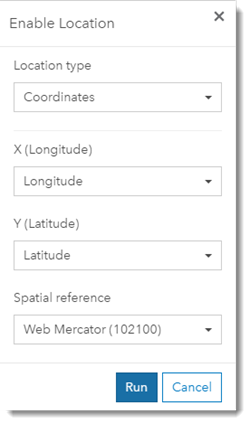The image depicts a webpage, primarily designed for mobile usage, prompting the user to enable location services. At the top, there's an "Enable Location" prompt with an adjacent close (X) button. Below this prompt, there's a section labeled "Location Type" displayed in a text box that reads "Coordinates." To the right of this, a drop-down menu is visible.

Following this, separate fields for "Longitude" and "Latitude" are displayed, each with corresponding drop-down menus. Both fields are filled, indicating longitude and latitude values. Below these fields, there is a section for "Spatial Reference," specifying "Web Mercator (102100)," also accompanied by a drop-down menu.

At the bottom of the webpage, there are two buttons: a blue "Run" button with white text on the left, and a white "Cancel" button with blue text and a blue outline on the right. The overall design is minimalistic, lacking distinct colors or identifiers to clearly indicate the website’s purpose, suggesting it might be part of a larger navigational or data entry process.